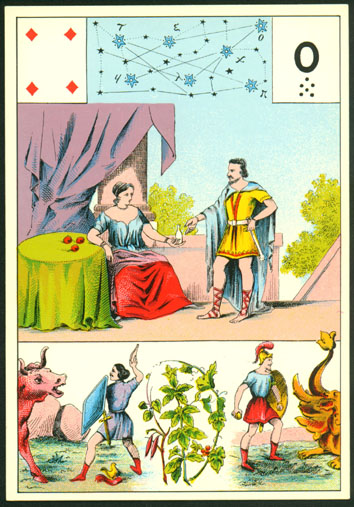This illustration appears to be a historical artwork composed of two distinct scenes, exuding an ancient aesthetic. 

At the top, we see an aristocratic man dressed in a yellow suit and blue cape, indicative of attire from centuries past. His attire includes a tunic and tied-on shoes, presenting a look reminiscent of medieval or Renaissance fashion. The man, sporting a mustache, gestures towards a seated woman at a table adorned with a green cloth and several apples. The woman faces him, extending a white bottle, while resting her other arm on the table. Behind the woman, a purple curtain draped over a column and lush green plants contribute to the scene’s depth. Above this interaction, a constellation-like arrangement of stars and letters offers a celestial touch. Additionally, the top left features a small white box with four red diamonds, and the right side presents another box with an 'O' or zero flanked by six points beneath it.

In the bottom image, two men are depicted in a stance that evokes action or confrontation. The man on the left, clad in a purple tunic, wields a blue shield and a sword, directing his attention towards a red bull accompanied by a small golden chicken-like creature at its feet. The man on the right dons a Roman-style helmet and holds a golden shield, positioned protectively in front of an indistinct golden animal. Between the two figures lies a green plant adorned with small red berries, heightening the sense of nature interwoven with the martial elements.

These detailed scenes are intricately illustrated, showcasing a blend of historical references, mythological elements, and rich symbolism.